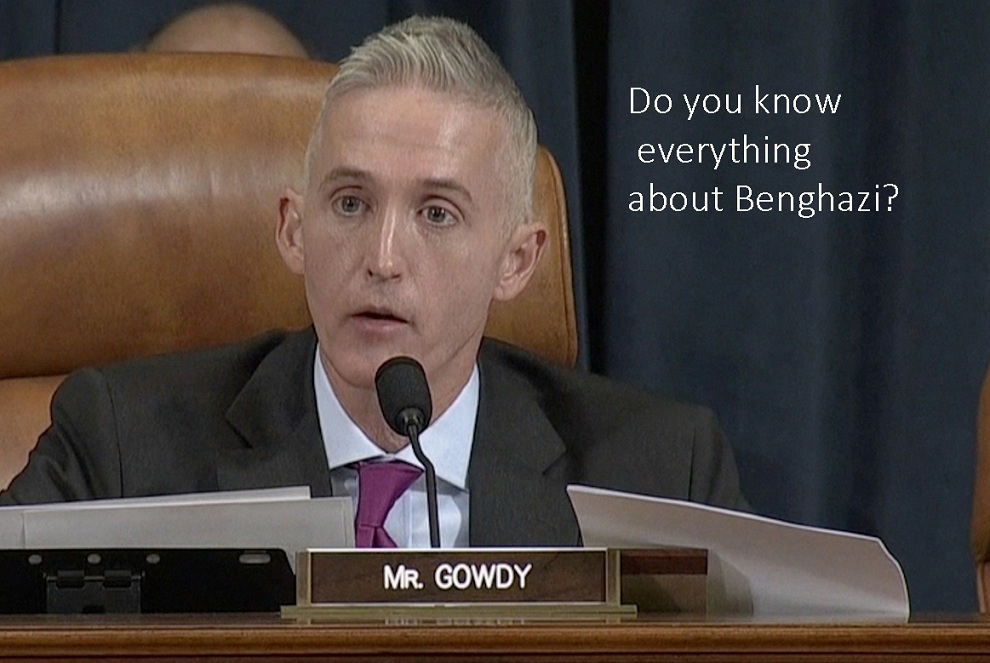In this photograph, former United States Representative Trey Gowdy is seated in a large, overstuffed light brown leather chair with a high back. He is dressed in a dark gray suit, complemented by a white button-down shirt and a magenta tie. Gowdy, a Caucasian male in his 50s, has very fair skin and short gray hair styled with gel, cut closely on the sides and spiked upward on top. The image captures him from chest level up to his head.

Gowdy is speaking into a thin black microphone positioned in front of him on a desk. On the desk are several papers and a tablet. Directly in front of him sits a wooden nameplate that reads "Mr. Gowdy" in white lettering. The background features a black curtain, and in the upper right corner of the photograph, white text reads, "Do you know everything about Benghazi?" This text partially overlaps the image, adding context to the setting, which appears to be a Congressional hearing or a similar formal setup.